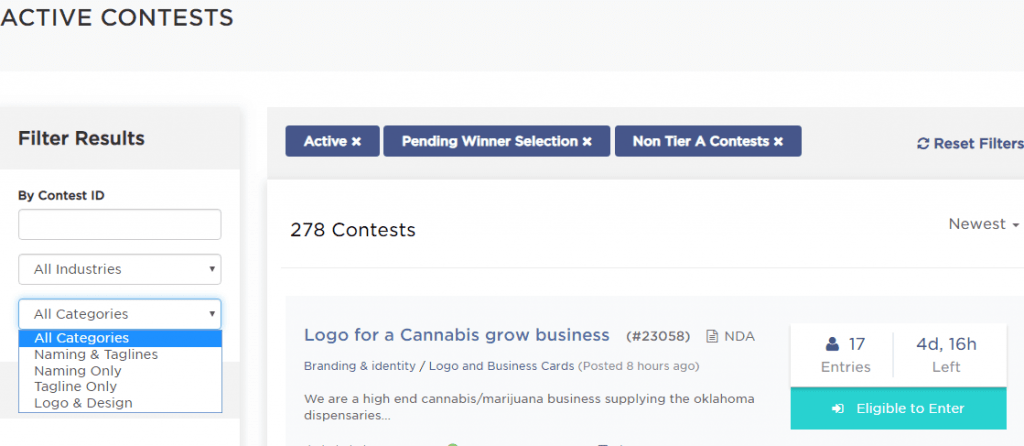This image is a detailed screenshot of an online platform showcasing a list of active contests. At the top of the screen, the heading "Active Contests" is prominently displayed. On the left side, there's a "Filter Results" section that offers several filtering options including contest ID, industry, and category. Additionally, there is a drop-down menu under "All Categories" which includes choices like "Naming and Taglines," "Naming Only," "Tagline Only," and "Logo and Design."

On the right side, the interface features various contest status tabs such as "Active," "Pending Winner Selection," "Non-Tier A Contests," with "Active" being the currently selected tab. Directly below these tabs, the platform indicates there are 278 active contests available.

One highlighted contest is titled "Logo for a Cannabis Grow Business" and is identified by contest ID number 23058. An NDA (Non-Disclosure Agreement) icon is visibly next to the contest title, indicating confidentiality requirements. This particular contest falls under the "Branding and Identity" and "Logo and Business Cards" category and was posted eight hours ago.

The website appears to be a platform where users can participate in various contests related to logo design, branding, and other creative endeavors for a chance to win. The detailed organizational structure and filtering options suggest a user-friendly experience for contest entrants.